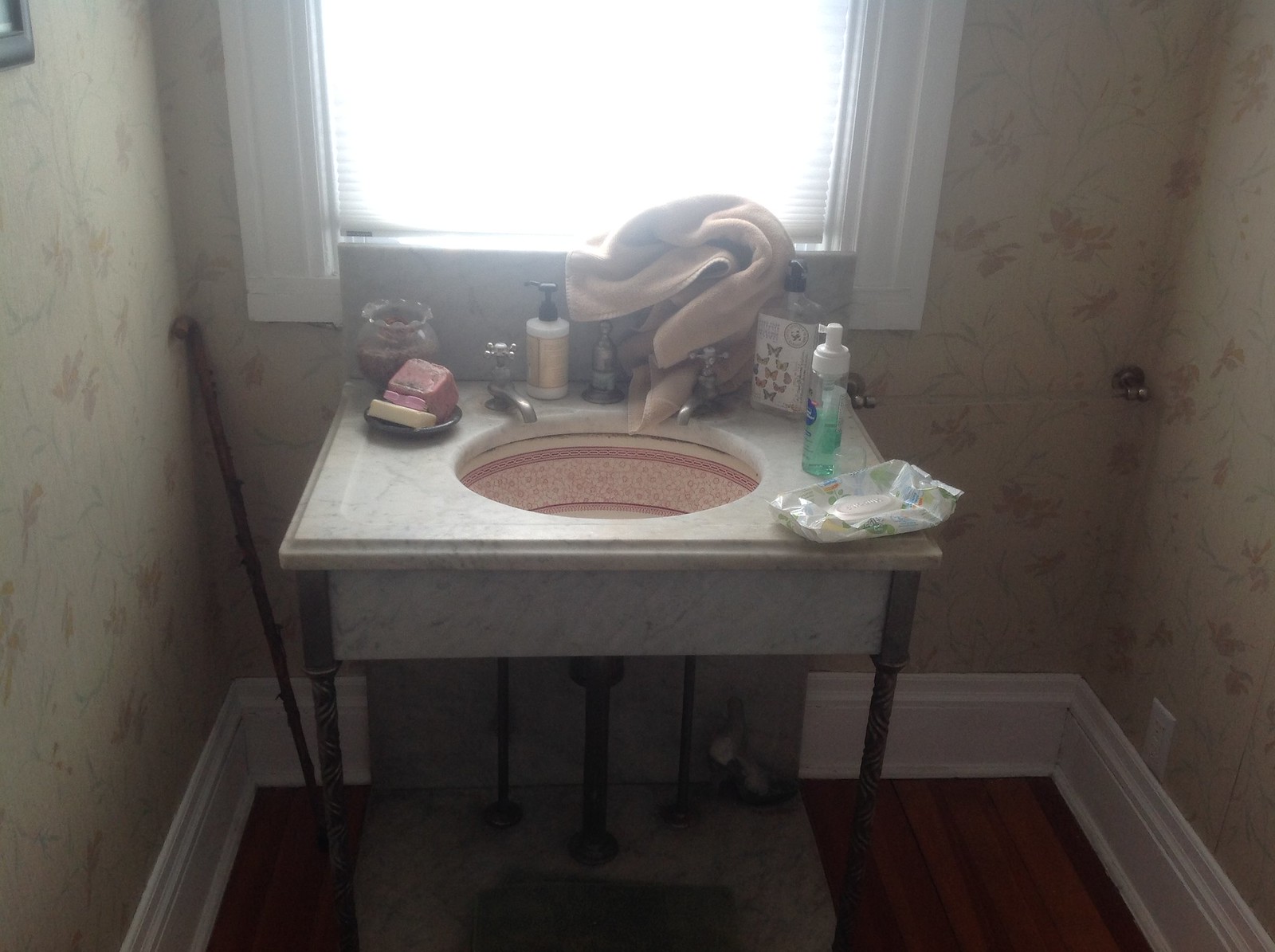This image captures a serene bathroom scene featuring a standalone porcelain white sink situated directly in front of a window adorned with light-filtering blinds. The window looks out onto a surface covered in white wood paneling. The walls are lined with beige wallpaper accented with dainty pink flowers, creating a soft, inviting atmosphere.

The sink rests atop a dark wooden floor, offering a striking contrast. On the sink’s edge, there's a neat tray holding a diverse collection of soaps, predominantly in shades of pink and white. Two gleaming silver faucets are installed on the sink. Draped over one faucet is a medium-sized hand towel. Next to the tray, a candle adds a touch of warmth and comfort, while a packet of wet wipes in a white wrapper teeters on the edge.

Among the essentials placed on the sink are a green hand soap dispenser and another decorative soap with intricate designs. Situated right behind one of the faucets is a small lotion dispenser. Adjacent to the sink on the right is a sleek silver towel bar, currently unused, lending a minimalist touch.

Toward the bottom left side of the wall, there's a white electrical socket, blending seamlessly with the white border skirting the floor, which ties the room together with a touch of classic detailing.